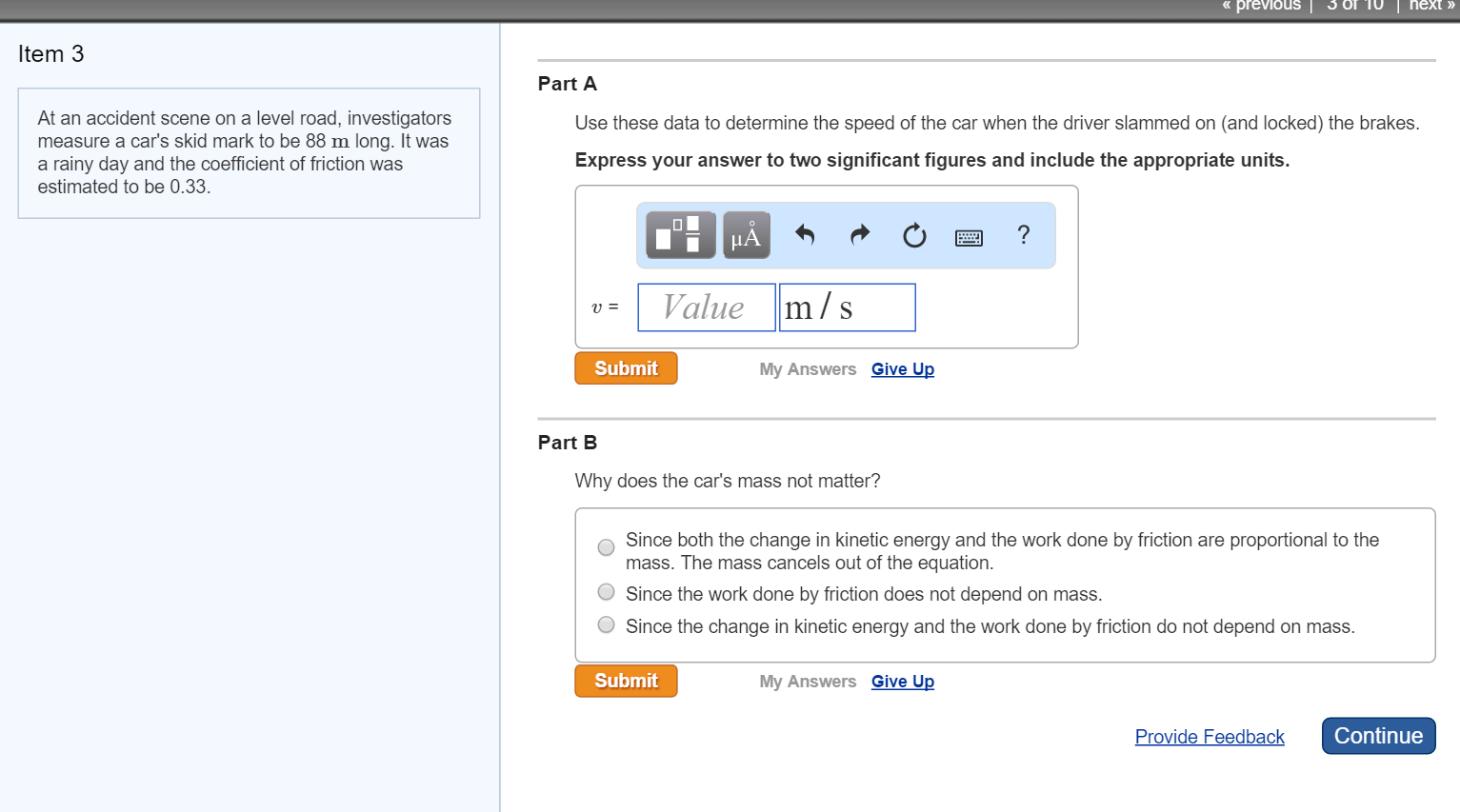The image appears to be a screenshot from a computer-based test or evaluation related to an accident scene investigation. The layout features a gray strip at the top right corner displaying navigation options such as "previous," "three of 10," and "next." Below this, the left side of the screen is colored in light blue and contains text labeled "item 3." The description details an accident on a level road where investigators measured a car's skid mark to be 88 meters long on a rainy day, with a coefficient of friction estimated at 0.33.

On the right side, the screen is white with black text divided into sections labeled "Part A" and "Part B." In Part A, users are instructed to use the given data to calculate the speed of the car when the brakes were applied, expressing the answer to two significant figures and including the appropriate units. This section includes interactive elements such as input fields for calculations, buttons for submitting answers, and options to view the answers or give up.

Part B prompts users to explain why the car's mass does not affect the calculation, with multiple-choice options and a circle to mark the correct answer. Similar to Part A, this section also features "submit my answers" and "give up" buttons. At the bottom of the screen, there are additional buttons for providing feedback and continuing to the next part of the test.